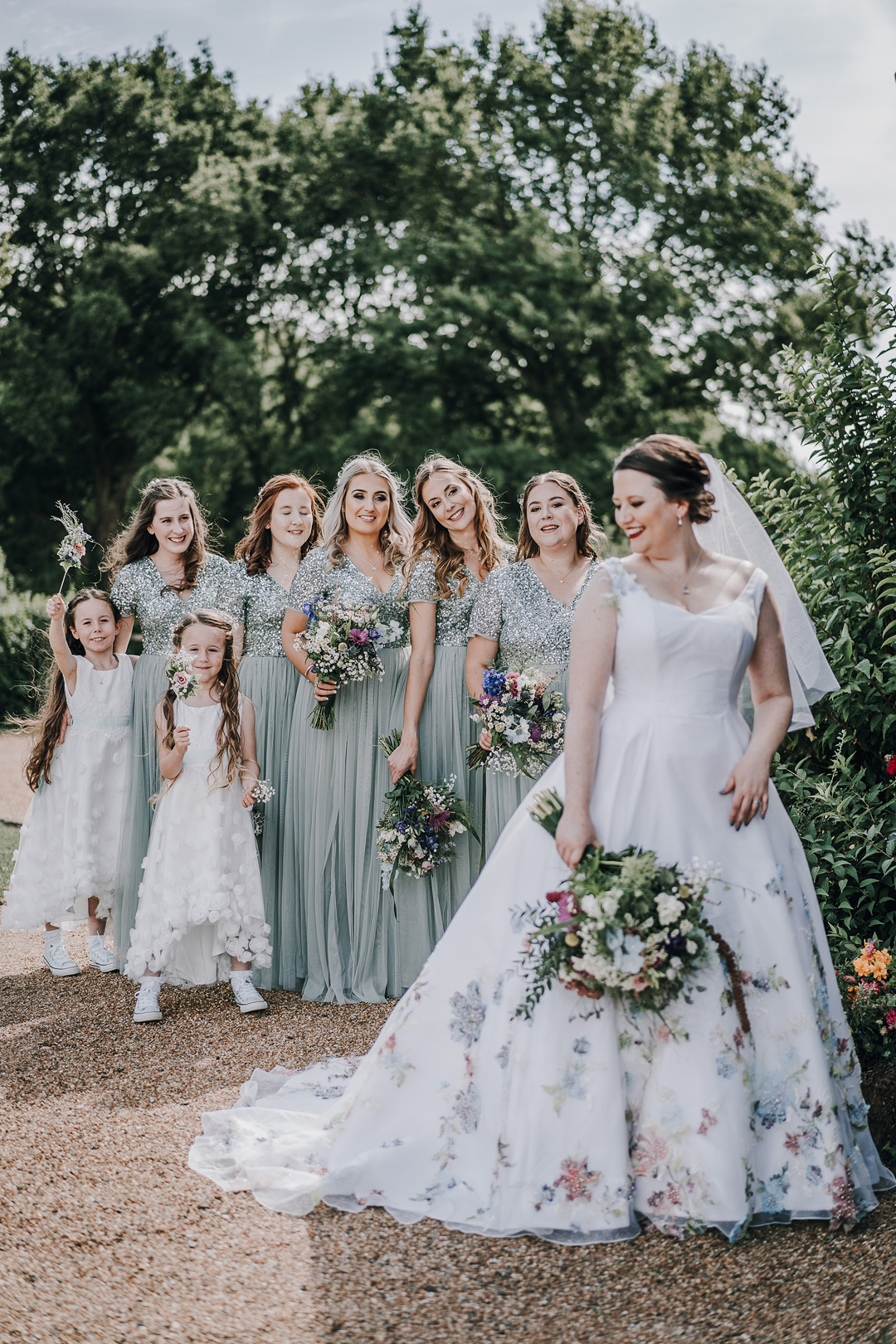In this vibrant outdoor wedding photograph, taken during the daytime under natural, dappled light, the focal point is the radiant bride standing on a gravel surface with a serene backdrop of green trees and sky. She wears a stunning sleeveless white dress with a sweetheart neckline and a wide bodice, elegantly embellished with colorful floral patterns at the hem. Her bouquet, held low, perfectly matches the floral detail of her dress. The bride’s hair is styled in a neat bun, adorned with a veil, and she casts a warm, pensive smile while looking down.

Surrounding the bride are five bridesmaids, each dressed in sage-green, floor-length gowns with short sleeves. Each bridesmaid holds a smaller bouquet that complements the bride’s arrangement. Positioned in front of the bridesmaids are two cheerful young flower girls in matching white dresses. The entire wedding party, composed of Caucasian individuals, is arranged on a brown pebbled ground, lending a rustic charm to the scene.

The photograph, captured in portrait orientation, showcases a sense of joyful celebration through its realistic and representational style, masterfully highlighting the harmonious blend of floral motifs and the natural beauty of the outdoor setting.